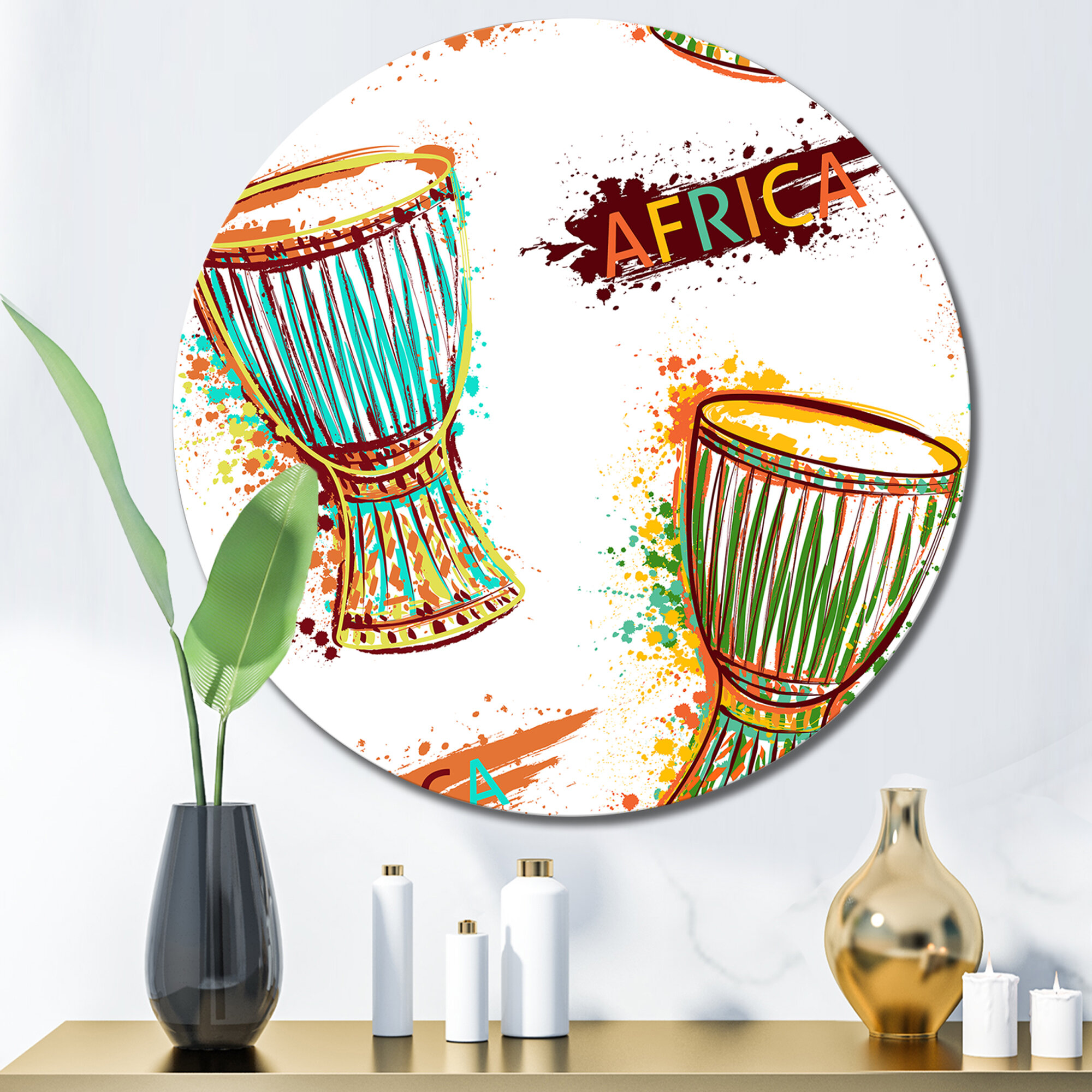This image features a seemingly rendered home interior. Highlighting the décor is a large, flat, circular Art Deco plate hanging on a white wall. The plate is predominantly white and vividly decorated with festive, colorful splotches of red, yellow, and blue paint, suggesting a celebratory theme. Painted on the plate are two elongated drums, similar to bongos. The drum on the right side is partially cut off and features an orange top with a blue and red body accented by gold trim. Below it, in the bottom left section of the plate, is the second drum, showcasing green and orange hues. The word "Africa" is prominently written to the left of the drums in brown lettering, with each letter of "Africa" colored differently: A is red, F is yellow, R is blue, C is yellow, and the final A is red.

Beneath the plate, a short tan table with a reflective, golden surface adds to the entryway's décor. Atop the table is a sleek black vase holding two large green leaves. Positioned next to the vase are three white bottles of varying sizes, all capped in gold. To the left, a gold vase stands beside two small, flameless white pillar candles, completing the arrangement. The combination of these elements creates a harmonious and lively atmosphere, blending art and functionality.